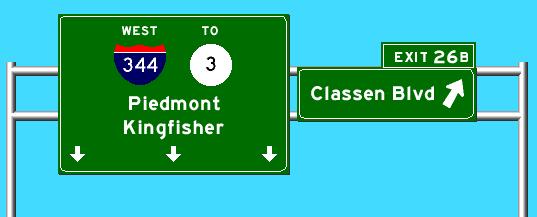This image appears to be a digital mock-up of an interstate road sign, likely designed for a mobile game or simulation. The backdrop is a blend of sea foam green and bright blue, simulating a clear sky. The signage is suspended on an arched metal frame consisting of two vertical metal poles on either side of a roadway, with two horizontal crossbars supporting the signs.

On the left, there's a large green rectangular sign that reads "West 344 to 3" with "344" displayed in a red and blue shield shape and "3" inside a white circle with green writing. The text "Piedmont Kingfisher" is prominently displayed below, accompanied by three downward-pointing arrows. To the right, another green rectangular sign reads "Classen Boulevard" with an arrow pointing up and to the right. Above this, a smaller sign specifies "Exit 26B." All signs feature white text and arrows, with the exception of the red and blue shield. The entire structure is held up by metallic, silver-colored poles, adding a realistic touch to the otherwise simplistic animation.